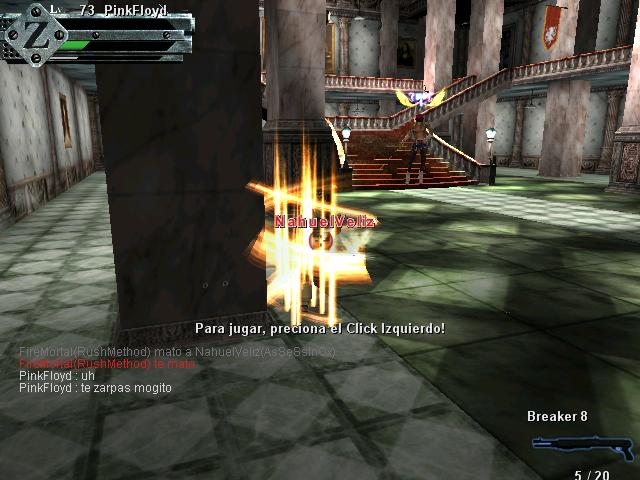In this image from a video game, the first floor of an expansive hotel or building is depicted, featuring a green carpet and a banner bearing various inscriptions in a different language. At the center of the scene, a character, possibly a woman with her hair pulled back, descends the staircase. The character appears to be wearing tight jeans and boots, but the exact details of the outfit are unclear.

The staircase, which is centrally located, does not ascend very far before it turns at a platform and continues to the second floor. On one of the walls hangs a notable banner featuring the text "73 Pink Floyd" in the upper left corner, alongside a large 'Z' on a metal plate and the phrase "Pink Floyd" repeated below. The banner also includes the phrase "Te Zarpas Maguito," which is not in English and whose meaning is unclear. Additionally, towards the lower right corner of the banner, the text "Breaker 8" and the date "5/20" can be seen, further adding to the enigmatic and atmospheric setting.